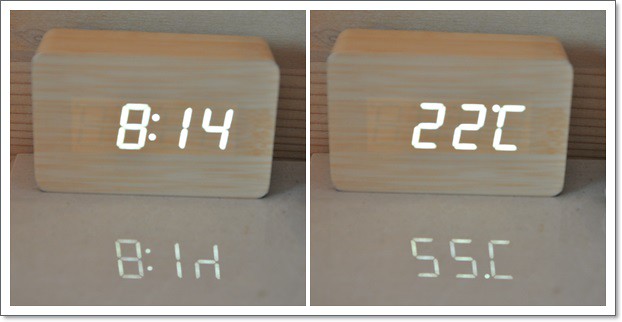The photograph is split into two individual images separated by a white vertical line, framed by a thin white border. The entire composition features various shades of tan and light brown, with both images presenting a brick-shaped object reminiscent of wood but likely made of plastic, showcasing a wood grain pattern. Each object is set against a tan background that could be a wooden shelf or surface.

On the left side, the object functions as a digital clock, displaying "8:14" in bright white LED numbers, with the time also reflected on the surface below it. The right side features the same visually identical object but in its role as a thermometer, displaying "22°C," also reflected on the surface beneath. The consistent reflection of the LED numbers in both images underscores the dual functionality of the product, suggesting it could be an ad highlighting its use as both a timer or alarm clock and a thermostat.